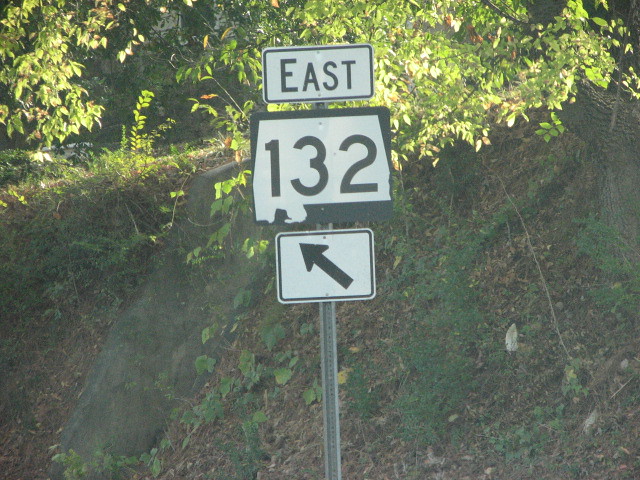The photograph captures a highway sign directing travelers along Pennsylvania Route 132. This sign features three distinct placards: the top placard reads "EAST," the center placard bears the number "132" overlaid on a possible silhouette of Pennsylvania, and the bottom placard displays an arrow pointing up and to the left, indicating a left-hand turn. The scene is set against an embankment adorned with vines, showing areas of visible erosion. Adjacent to the highway sign is a concrete-lined spillway cascading down the embankment. The presence of young shoots and fresh leaves suggests that the photo was taken in the spring. The sunlight filters through the foliage, casting a gentle glow on the simple yet functional signpost and its surroundings.